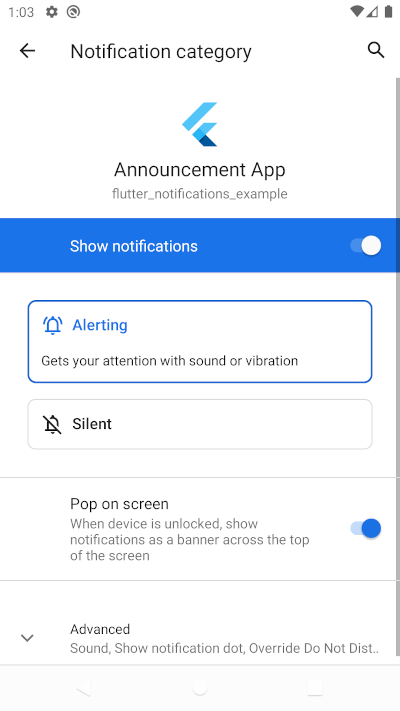This screenshot, captured from a cell phone, displays the "Notification Category" screen. On the top-left corner is a back arrow; to its right is a magnifying glass icon. Below these icons, prominently centered, is a logo resembling a stylized 'F'. The logo is tilted left with the bottom pointing to the bottom right. The design of the 'F' includes a light blue top and bottom horizontal bar, while the vertical leg is a dark blue.

Underneath the logo, the text "Announcement App" is prominently displayed. Below this, the option "Show notifications" is visible and toggled on. Further down, there is an "Alerting" category, which is indicated by a square with a thin blue outline. Adjacent to this, the "Silent" option is displayed. At the bottom, the "Pop on screen" option is also visible and toggled on.